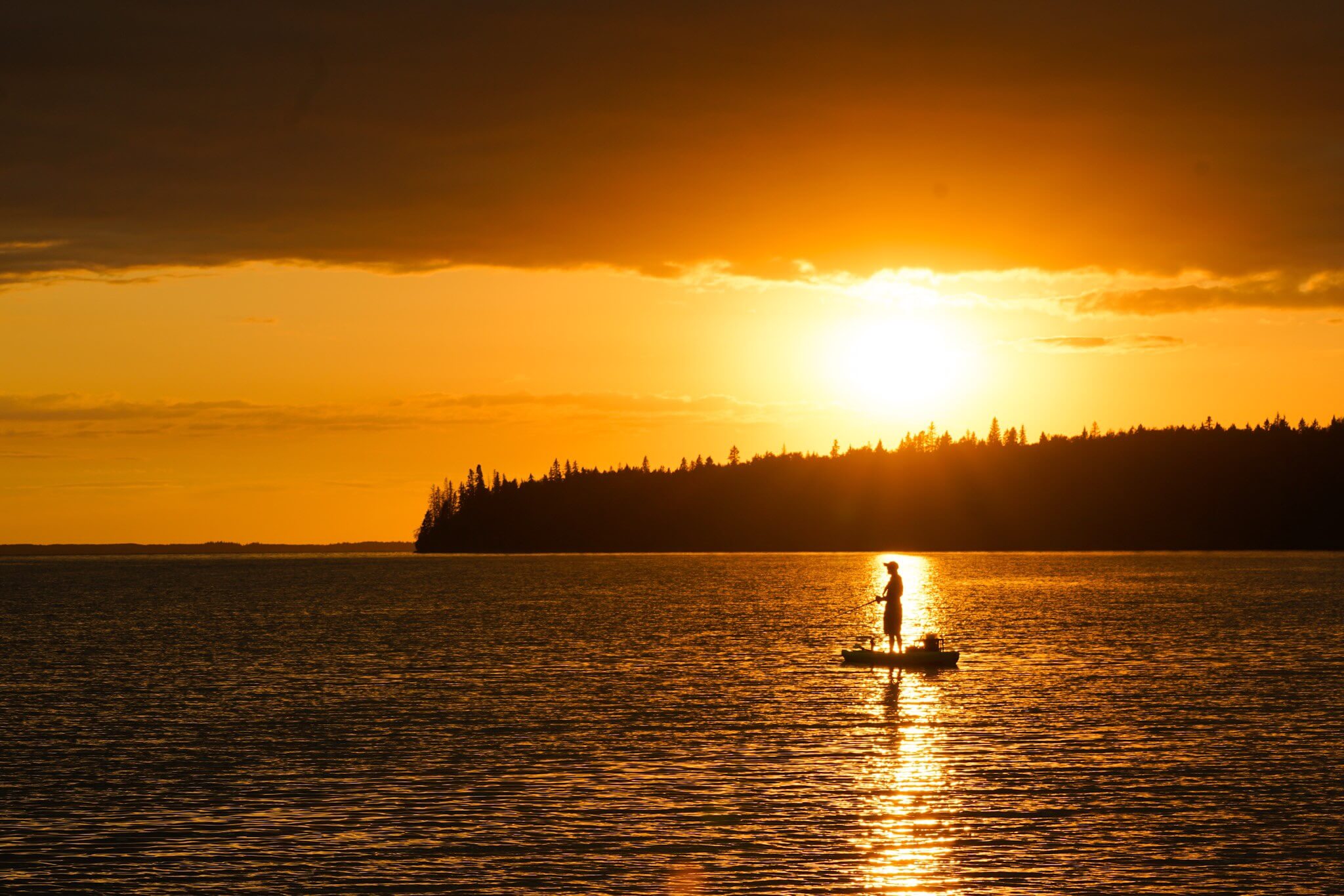A captivating image reveals a silhouetted man standing upright on a small boat, likely a kayak, immersed in the peaceful act of fishing as the sun sets behind him. The scene, awash in a dramatic palette of oranges and blacks, prominently features the sunset's reflection on the expansive body of water, contrasting strikingly with the darkened figure of the man holding a fishing rod and wearing a baseball cap. The calm water, with gentle ripples, extends toward a distant shoreline adorned with tall pine trees and an undisturbed wooded environment, devoid of any buildings or houses. The sun, large and glowing yellow with an orange halo, hangs low on the horizon, partially obscured by clouds that cover much of the upper sky, enhancing the serene yet vibrant ambiance of the moment.